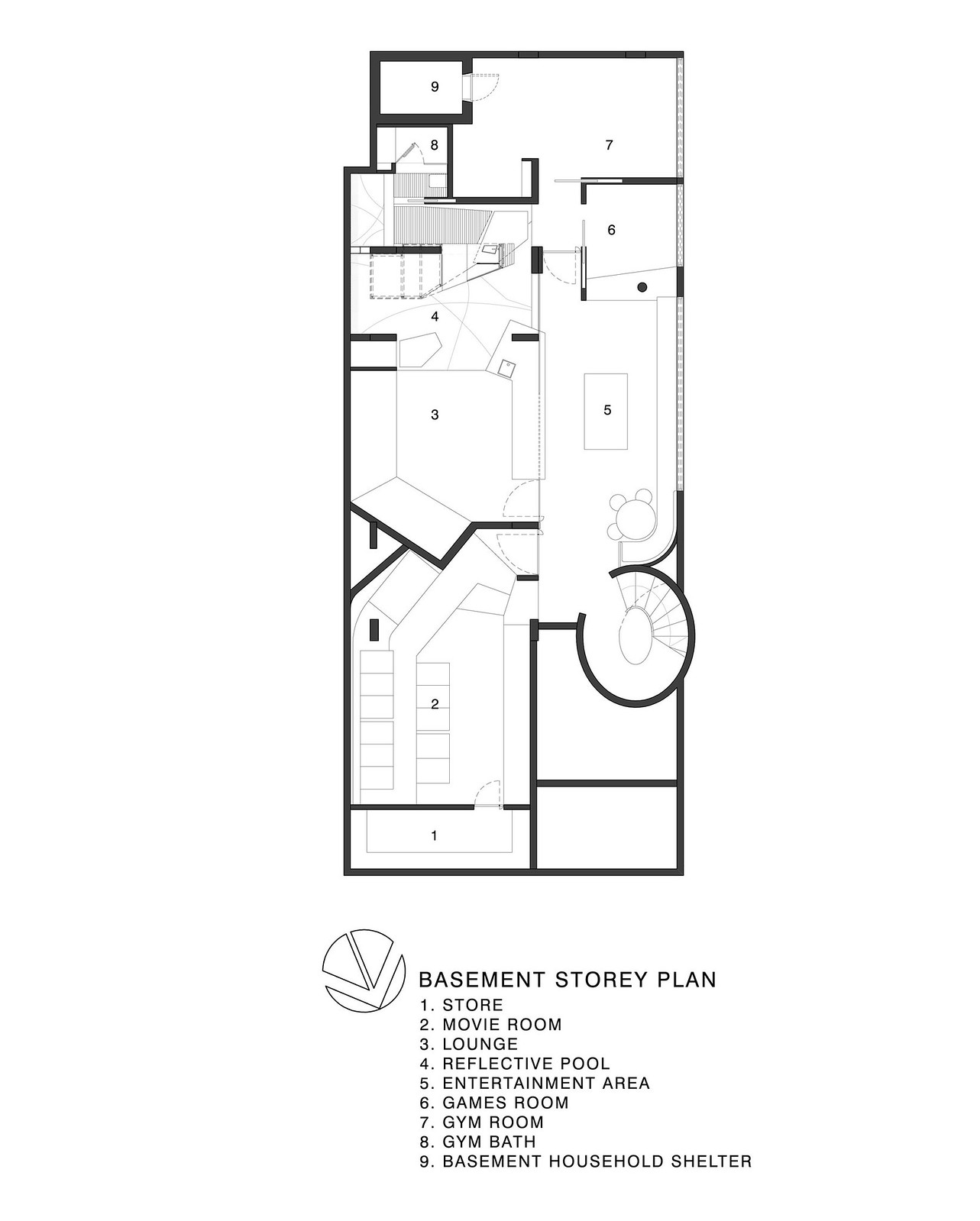This black-and-white photograph showcases a detailed blueprint of the basement level of a house. The blueprint is marked with a numerical legend from one to nine, identifying various rooms and areas within the basement. The layout features two sets of stairs—one a traditional staircase for regular access, and the other a spiral staircase, likely serving both aesthetic and functional purposes. 

Room annotations on the blueprint include:
1. A store room
2. A movie room
3. A lounge
4. A reflective pool
5. An entertainment area
6. A games room
7. A gym room
8. A gym bath
9. A basement household shelter

The household shelter, indicated with noticeably thick walls, suggests this area might be designed to serve as a secure space, possibly for emergencies such as tornadoes. The reinforced walls, appearing to be about a foot thick in the overhead view, reinforce this idea. 

This basement plan appears to be designed as the recreational and functional hub of the house, encompassing entertainment, fitness, and safety needs efficiently.